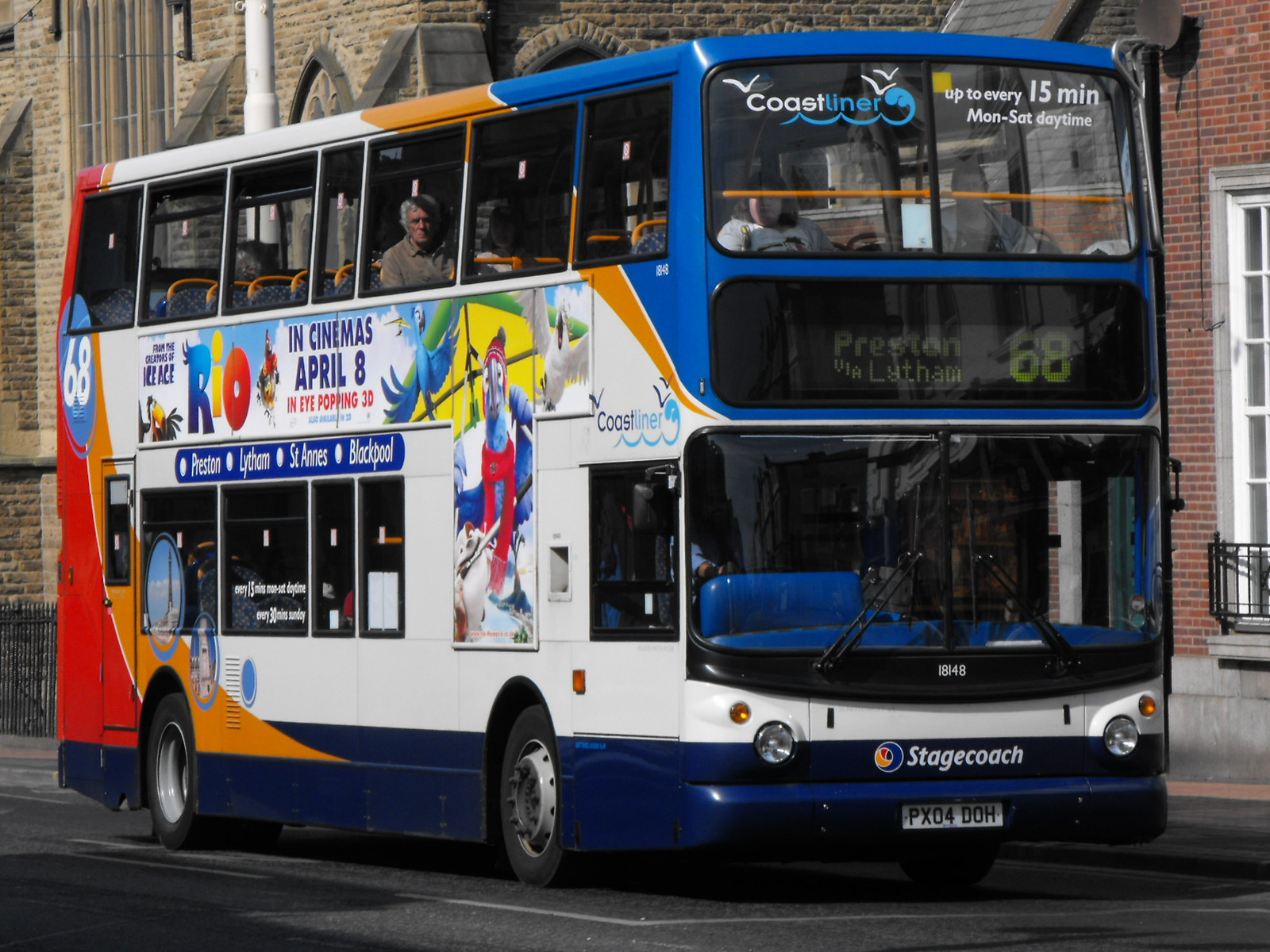This horizontal rectangular photograph captures a vibrant scene featuring a colorful double-decker bus parked on a city street against a backdrop of two distinct buildings. The bus, predominantly white with a blue front, blue bottom, and orange and red toward the back, boasts a lively advertisement reading "Rio in Cinema's April 8th in eye-popping 3D." The side also displays the destinations "Preston, Lytton, St. Ann's and Blackpool," alongside the bold "Coastliner" branding announcing service every 15 minutes from Monday through Saturday daytime. The bus features two levels with passengers seated on the top section, where the driver is also located. Handsome details like the license plate PX04DOH and the "Stagecoach" logo at the front further accentuate its character. The street is framed by a strong contrast of dark pavement and the two buildings: A probable church with rounded windows on the left and a standard red brick structure on the right. These elements come together to create a vivid urban tableau.